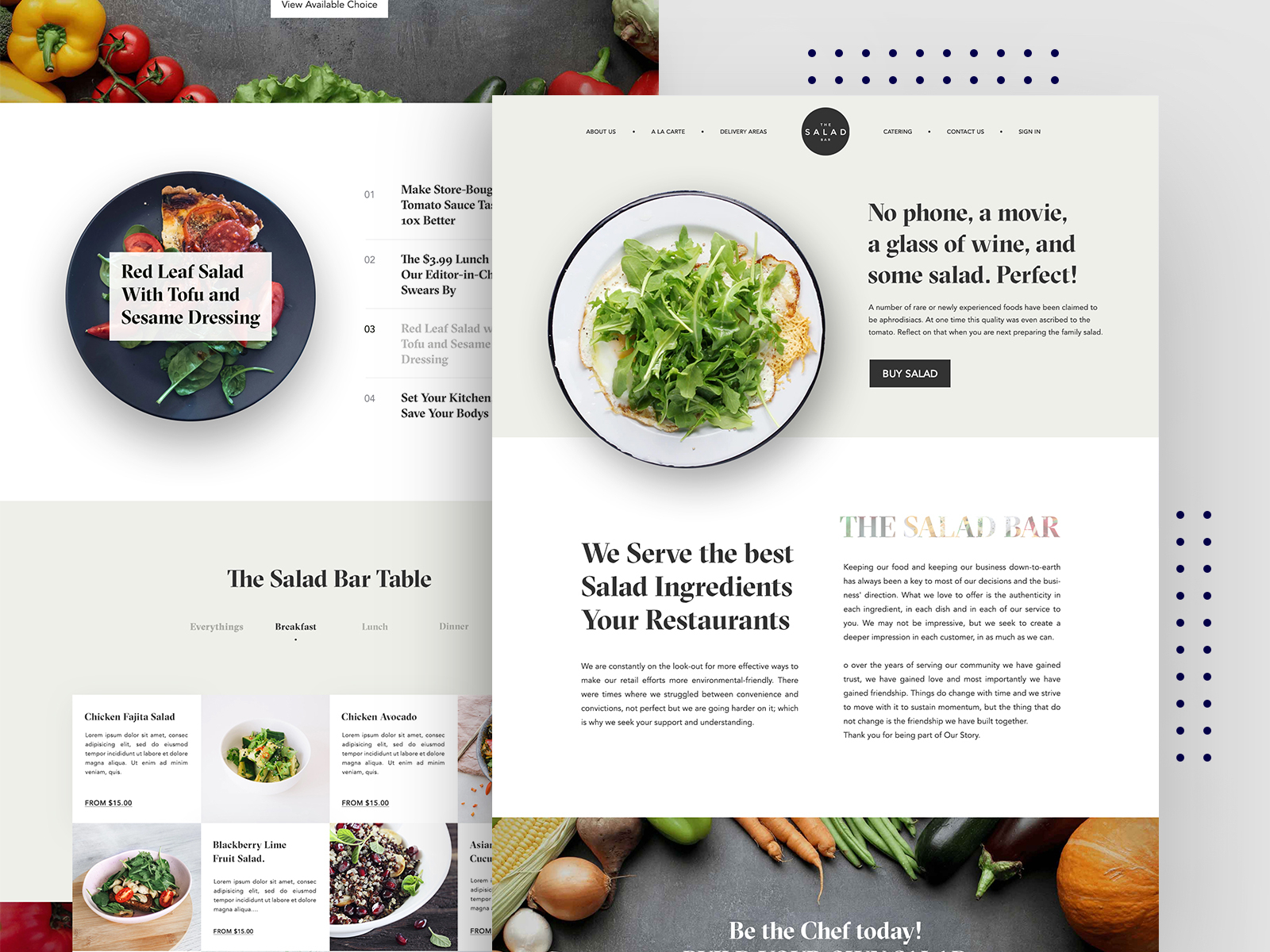The image appears to be a screenshot of a webpage featuring a grayish background. In the top left-hand corner, there's a gray banner adorned with vibrant images of various foods: yellow peppers, red tomatoes, green lettuce, and a few other colorful peppers towards the right side.

The top right-hand corner displays two rows of ten black dots each, a mirrored arrangement seen in the bottom right-hand corner where two columns of ten black dots reside.

Centrally placed is a gray pop-up box, bifurcated into two sections. The upper section, hued in light gray, contains the text: "No phone, a movie, a glass of wine, and some salad. Perfect." This text is complemented by a sentence in smaller font below: "A number of rare or newly experienced foods have been claimed to be aphrodisiacs. At one time, this quality was even ascribed to the tomato, reflecting that when you were next preparing the family salad."

Beneath the text, a black button prominently displays the phrase "Buy Salad."

Adjacent to this, an image shows a white plate garnished with fresh green leaves and drizzled with dressing. Under the image, bold black text proclaims, "We serve the best salad ingredients, your restaurants." A more detailed description follows below this statement.

On the left-hand side of the webpage, one can observe a darker gray plate brimming with fresh spinach leaves, red tomatoes, and possibly a quiche. Text within a box above this setup reads, "Red leaf salad with tofu and sesame dressing." At the bottom left, additional salads are displayed under the heading "The Salad Bar Table," accompanied by more images of appetizing salads.